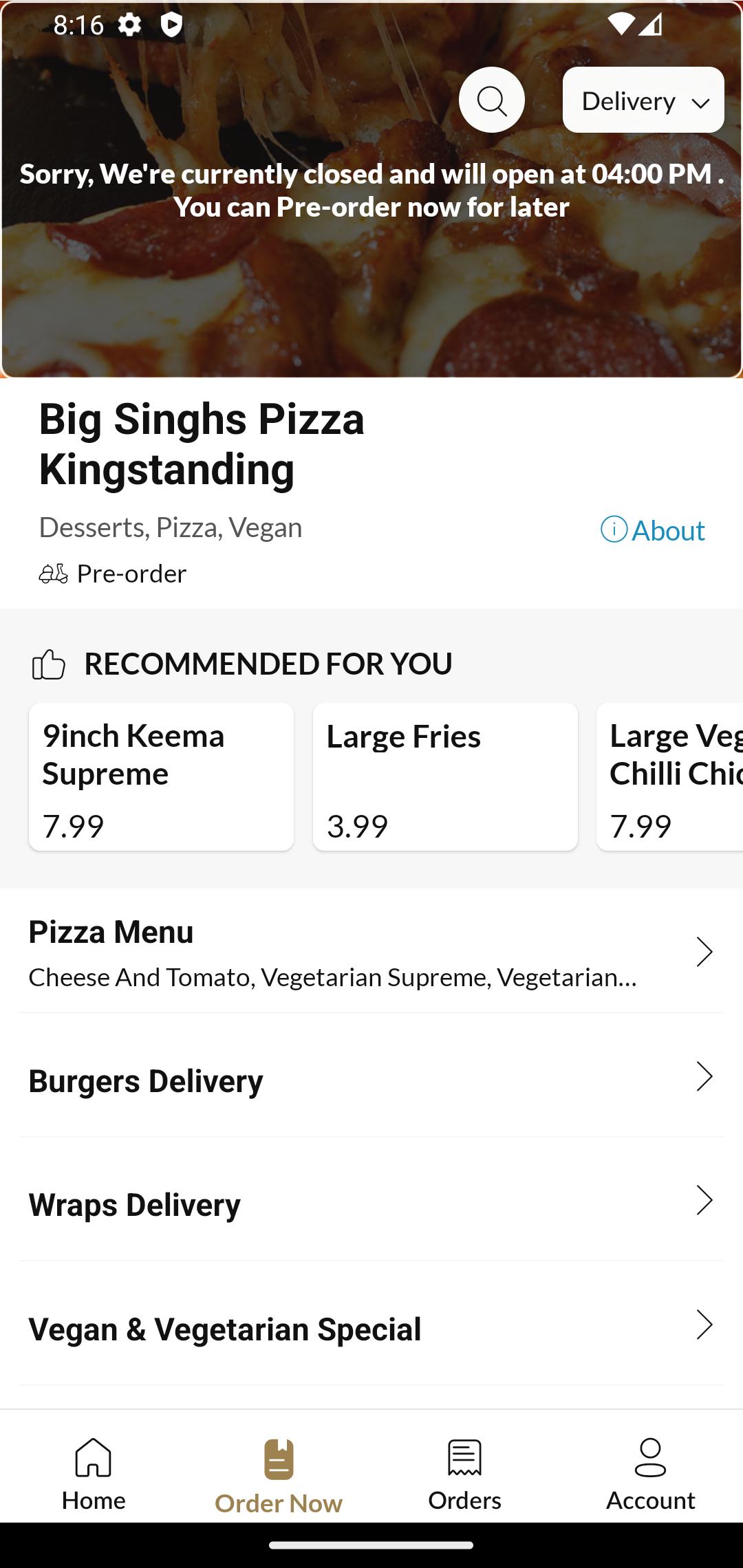This screenshot displays the homepage of a restaurant website, specifically for "Big Sings Pizza, King's Standing." At the top of the page, there's a header image showcasing a appetizing pizza. In the top right corner of the header, a magnifying glass icon is enclosed in a circle, symbolizing a search function. Adjacent to it is a notification box with the word "Delivery" and a message stating, "Sorry, we're closed. We're currently closed and we will open at 4pm." It also mentions, "You can pre-order now for later."

Below the header, on the left side, the restaurant’s name, "Big Sings Pizza, King's Standing," is prominently displayed. This is followed by menu categories for "Desserts," "Pizza," and "Vegan" options. On the right side of the page, there is an "About" link accompanied by an eye icon, and beneath it, a section titled "Recommended for you." This section lists menu items with associated buttons for quick ordering, including a "9 Inch Kima Supreme" priced at $7.99 and "Large Fries" for $3.99.